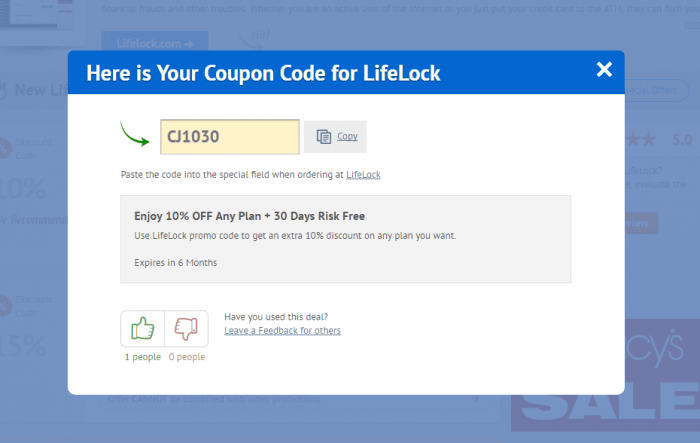Here is a detailed descriptive caption for the image:

---

The screenshot displays a pop-up window overlaying a blurred and indistinct background. The content of the pop-up window provides a promotional offer for LifeLock, presenting a coupon code "CJ1030" in bold text. A green arrow curves downward, directing attention towards the coupon code. Instructions indicate to copy and paste the code into the designated field when making a purchase on the LifeLock website to avail a 10% discount on any plan, along with a 30-day risk-free trial. The offer is valid for six months from issuance.

Below the promotional message, there are interactive elements showing a thumbs-up and thumbs-down icon. The thumbs-up icon has a tally indicating that 1 person has upvoted the deal, while the thumbs-down icon shows 0 downvotes. 

Additionally, there is a prompt asking users, "Have you used this deal?" with an invitation to leave feedback for others. This text is underlined, indicating it is a hyperlink that navigates users to a feedback page.

Notably, the image lacks any photographic elements or illustrations depicting people, animals, plants, buildings, bridges, or automobiles.

---